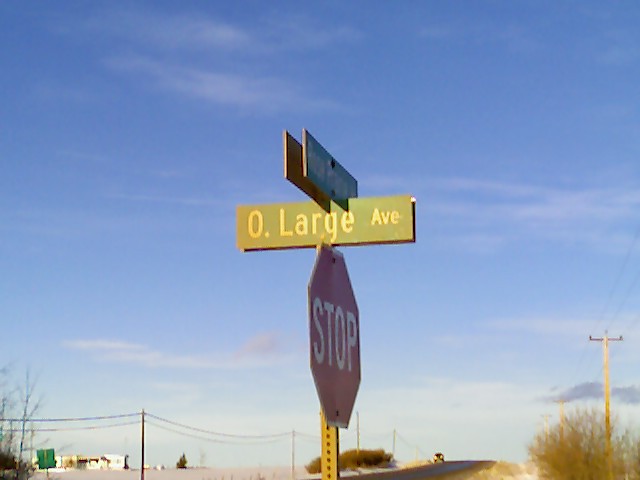Capturing a cinematic view of a street sign intersection, this image features a prominent stop sign at the forefront. Affixed to the top of the stop sign are two street name signs, arranged in a slightly crossed fashion. The sign directly facing the camera clearly displays its street name, while the one angled to the right is only partially visible from this perspective. Behind this top sign, there appears to be a duplicate facing the opposite direction, ensuring visibility from multiple angles. The stop sign itself is oriented towards the right side of the image, adding a sense of direction and guiding focus within the frame.